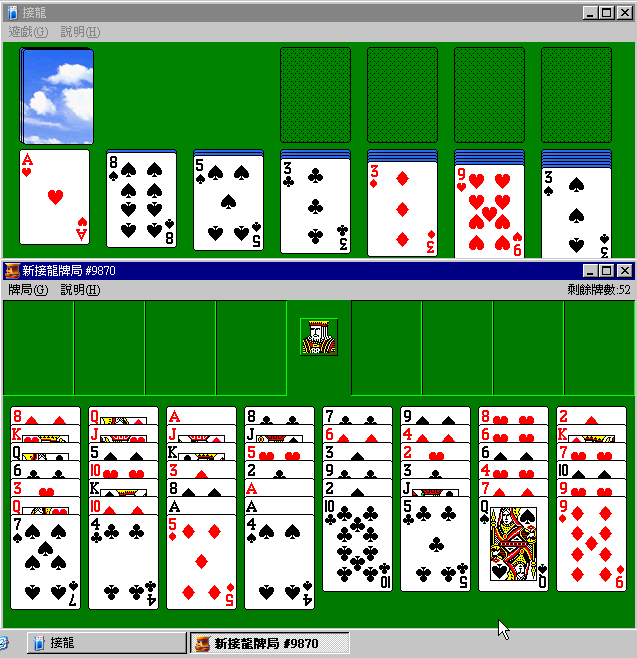In this screenshot of a virtual solitaire game, a player is engaged in a standard game of Solitaire, meticulously laying out cards on a green felt table simulated by the game's interface. The visual setup includes seven neatly organized columns of cards, each revealing several playable options. The game interface is presented in Asian characters, adding an intriguing linguistic element, though the exact language remains unidentified.

Within the tableau, we notice several intriguing openings: slots for a red 6, a red 3, a black 4, another red 3, and a red 9 among other potential moves. It is evident that the player has carefully set up multiple strategic options to continue advancing in the game. Overall, the setting is tidy and the cards are positioned with precision, enhancing the visual orderliness of the scene.